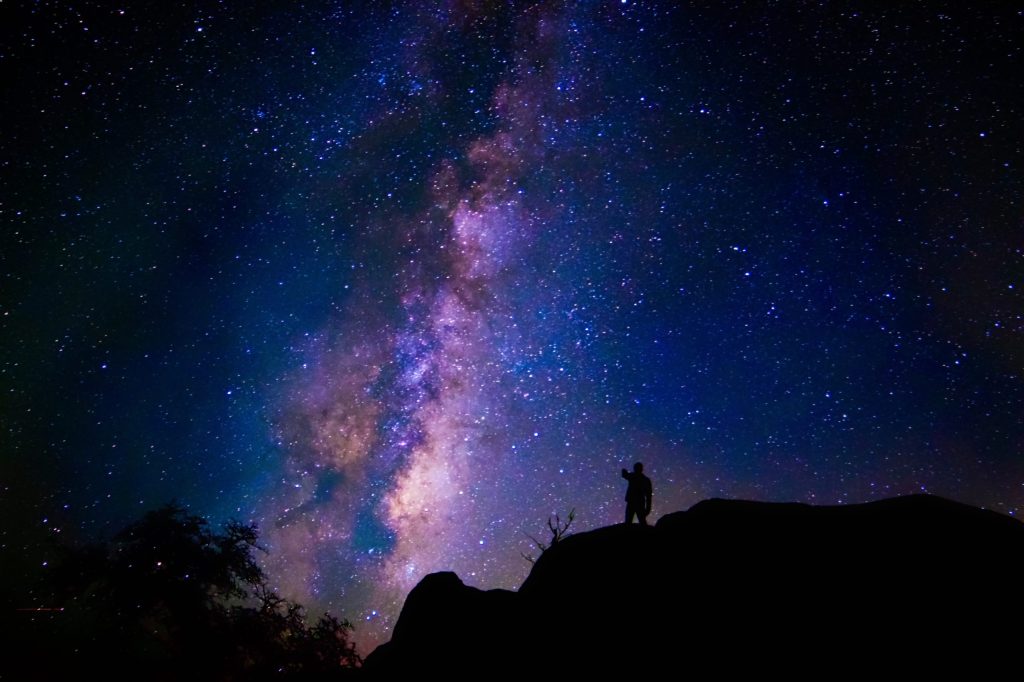This breathtaking image captures a mesmerizing night sky awash with hues of blue, purple, and mauve that seamlessly blend into the blackness around the edges. At the lower right-hand side of the scene, the striking silhouette of a rugged rock mountain comes into view. Atop this mountain stands a man, his darkened figure outlined against the sky, pointing upwards at the celestial wonder above. A small tree extends from the rock, adding another layer of contrast and depth. The sky itself is a spectacle, seemingly imbued with the colorful glow reminiscent of the Aurora Borealis, with countless stars dotting the expanse. There is a particularly captivating celestial body—perhaps a galaxy—emanating fiery reds to deep purples, standing out brightly amid the constellations. Additionally, on the left side of the image, the detailed silhouette of a large tree adds a further dimension to this enchanting nighttime tableau. The entire scene is imbued with a sense of cosmic wonder and beauty, making it a truly captivating sight.